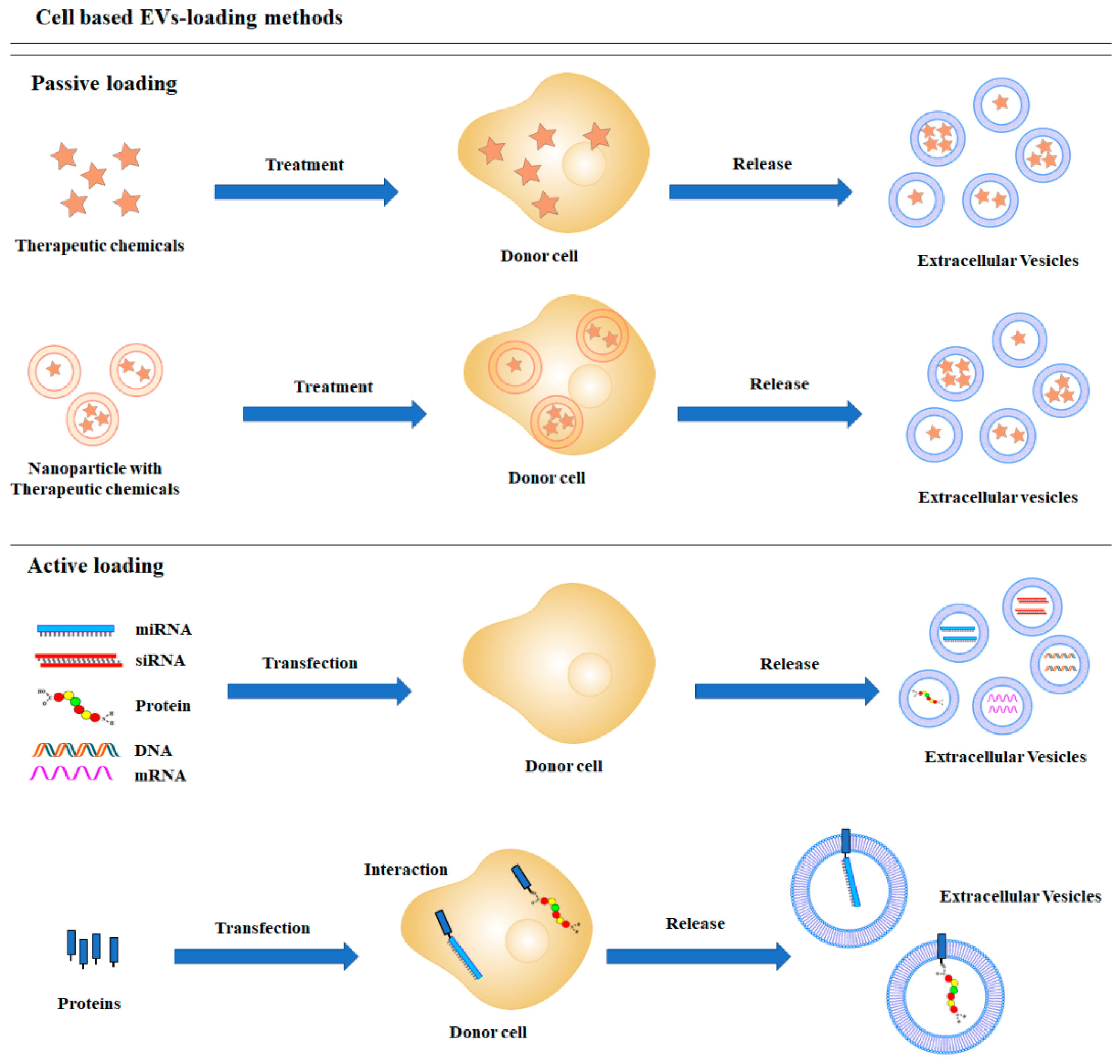This detailed image from a scientific or medical reference illustrates various cell-based extracellular vesicle (EV) loading methods. The diagram is divided into sections labeled "Passive Loading Methods" and "Active Loading Methods."

In the "Passive Loading Methods" section:
1. The first method involves therapeutic chemicals, represented by five orange stars. These stars are initially grouped together, followed by a blue arrow labeled "treatment," directing toward a donor cell depicted as a light gold circle containing the five orange stars. Another blue arrow labeled "release" leads from the donor cell to several extracellular vesicles (EVs) composed of differing numbers of stars within blue circles: one with four stars, one with three stars, two with one star each, and another with two stars.
2. The second method features nanoparticles containing therapeutic chemicals. These are represented similarly by stars in varying quantities (one to three) within orange circles. These are followed by a blue arrow labeled "treatment," leading to a donor cell depicted as a large orange circle containing these nanoparticles. A subsequent blue arrow labeled "release" directs to similarly labeled EVs as in the previous method.

In the "Active Loading Methods" section:
1. Different biomolecules are represented: blue lines for mRNA with hanging strands, red strands with lines in between for siRNA, a red, yellow, green dotted line for proteins, a squiggled orange and blue line for DNA, and irregular pink lines for other forms of RNA. These are used for transfection, indicated by a blue arrow pointing to a donor cell. 
2. This donor cell is depicted again as a light gold shape with these biomolecules inside it. Another blue arrow labeled "release" leads to EVs, showing various configurations: one with a square containing red, yellow, green, and blue dots, and another with a longer blue rectangle connected to a dark blue square.

The image systematically details cell-based EV loading methods, highlighting the progression from initial therapeutic substances to donor cells and final EV release, all indicated through color-coded arrows and specific representations of chemical compounds and biomolecules.